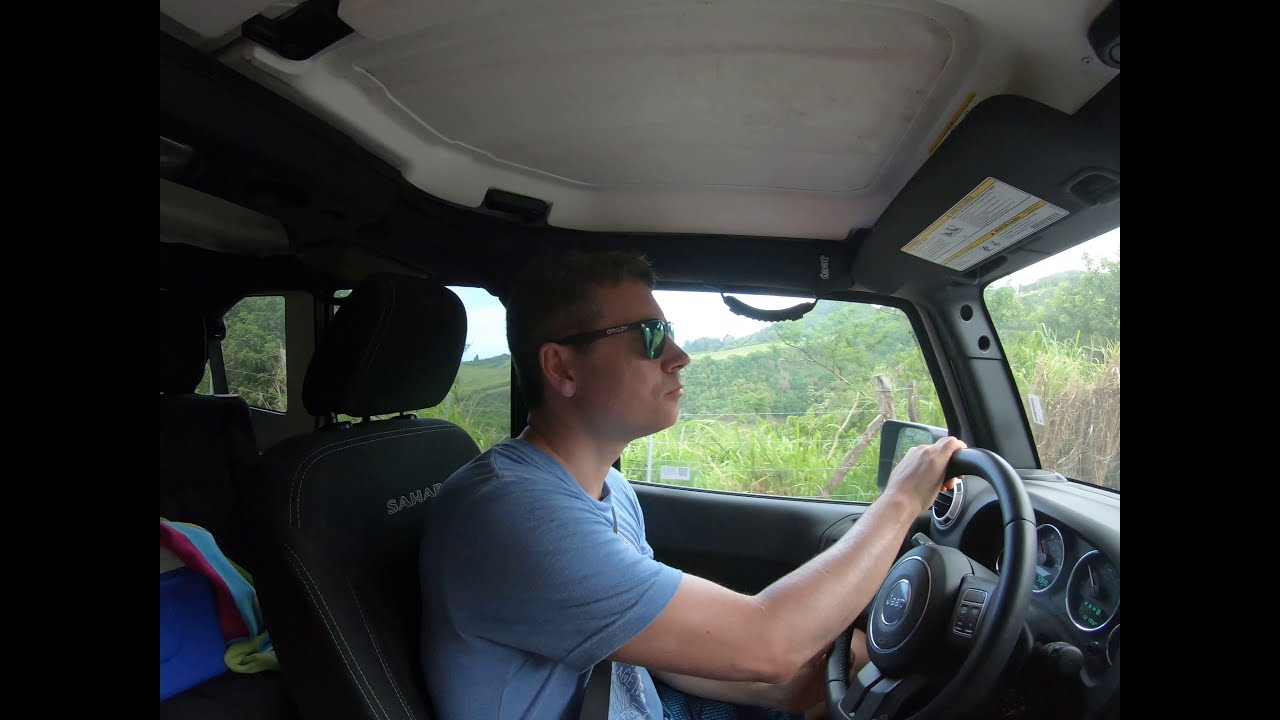The image captures a man driving a vehicle, likely an SUV, with distinct vertical black bars framing the left and right edges. The man, who is Caucasian with short hair, is seen facing the right, wearing sunglasses and a light blue short-sleeved t-shirt. His left hand grips the steering wheel while he looks ahead. The vehicle's interior features black seats and a white roof, which appears to be convertible. Text is faintly visible on the driver's seat, possibly reading "Sarum." Behind him in the back seat, there's a red, white, and green blanket or towel placed on what seems to be a blue cooler. Through the driver's side window and windshield, a scene of dense greenery unfolds, revealing a prairie landscape with a mix of tall grass, weeds, small trees, and a wire fence. In the distance, hills rise under a clear, daytime sky.